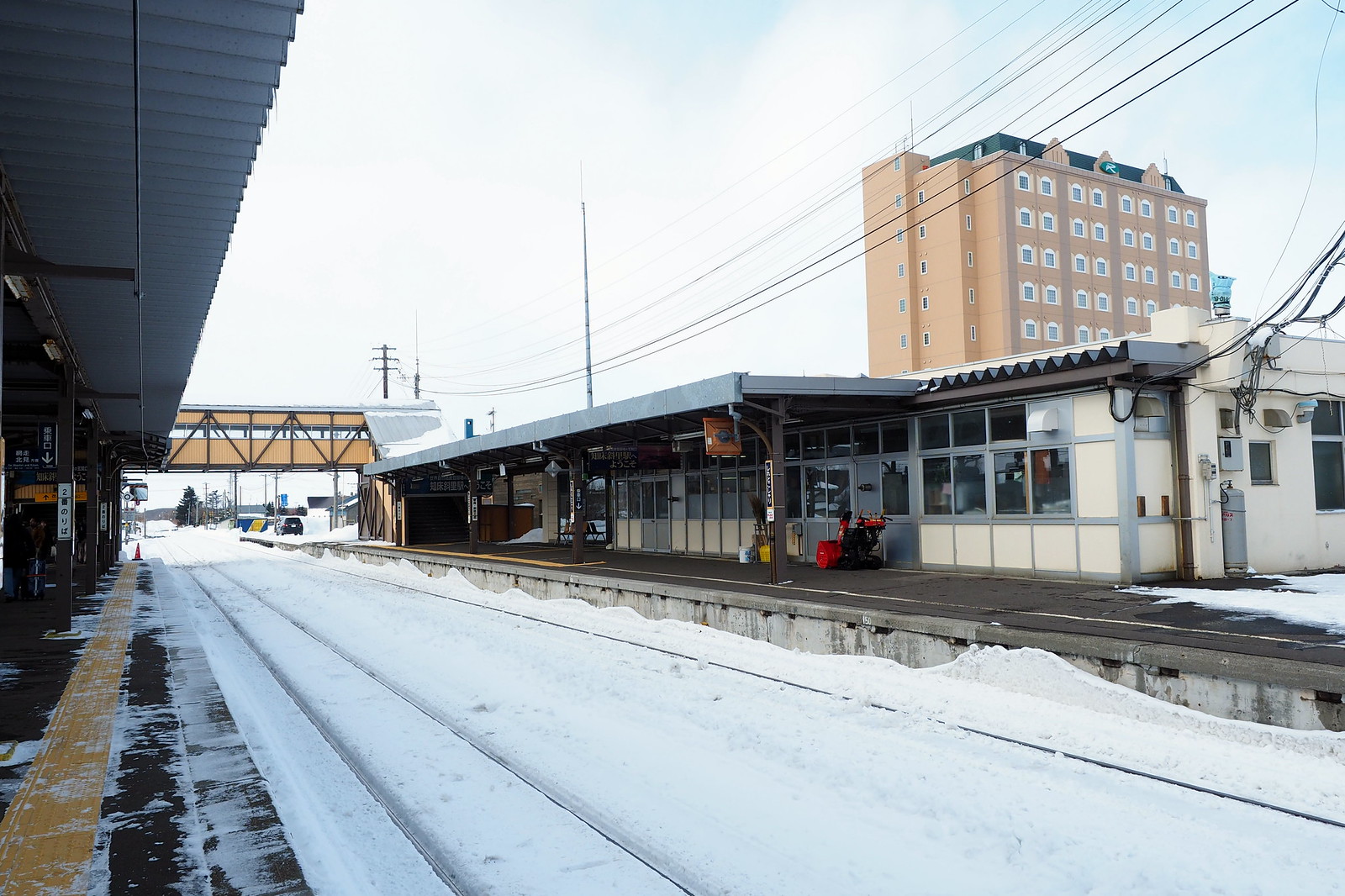A digital photograph captures a snow-covered train station. The scene is blanketed in white powdery snow, with the railroad tracks nearly buried beneath it. The station features a long white and blue building with numerous windows resting on a gray sidewalk pavement platform, which remains clear of snow. On both the left and right sides of the tracks, station platforms extend, even showing snow accumulation on their edges. Overhead, telephone towers and cables stretch across the right side of the station, and a zigzag-patterned bridge in the distance crosses over the tracks, providing passage between platforms. A prominent feature in the background is a large, brown apartment building with many white windows. The vivid colors of the scene include white, black, silver, gray, yellow, orange, tan, and teal, adding depth and contrast to the tranquil winter landscape.